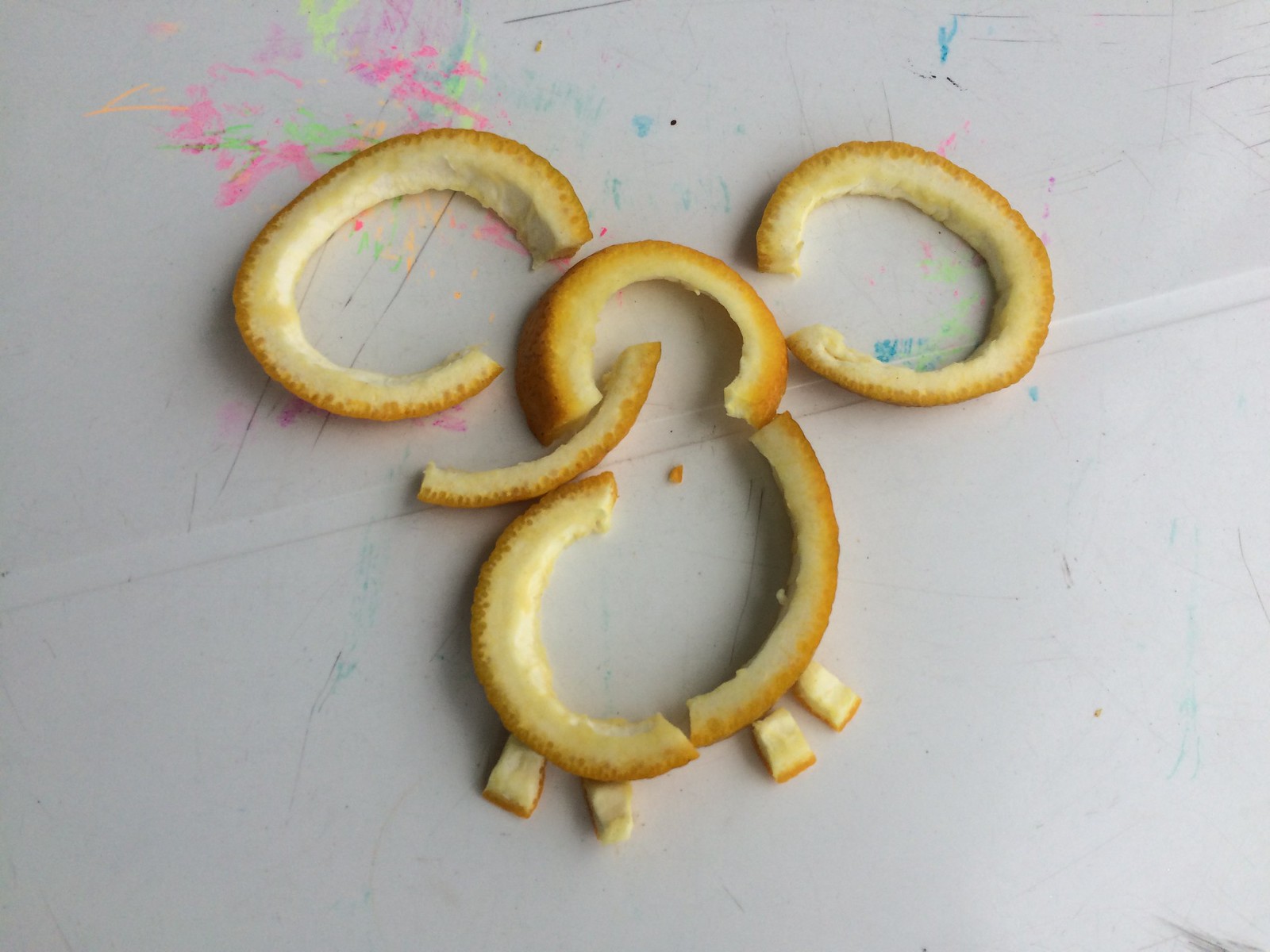The image showcases a creative arrangement made from orange peels, intricately assembled to form a whimsical figure that resembles a cross between an elephant and a Mickey Mouse character. The figure features two large circular peels for ears, smaller segments for legs, and a curved peel forming the trunk or mouth. This playful sculpture rests on a white surface, possibly an old art table, adorned with colorful, abstract splotches and scribbles of neon pink, blue, orange, green, and yellow, suggesting a child’s creative space. The background is marked with creases and hints of other artistic activities, hinting at a vibrant, imaginative setting.